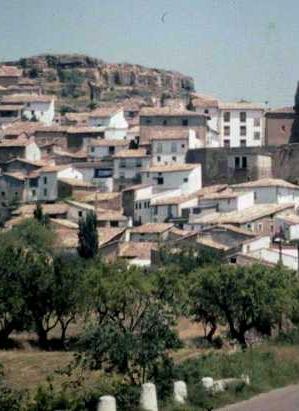This image captures a scenic, somewhat nostalgic view reminiscent of the 1970s, set in the Hollywood Hills. The picture showcases a collection of pristine white buildings with tan, brown-colored roofs and varying numbers of stories, nestled chaotically yet beautifully on a steep hillside. The houses, well-maintained and sophisticated, evoke an air of vintage luxury. In the foreground, lush greenery with densely populated trees and patches of green and brown grass frame the lower part of the scene. A small strip of gray roadway or trail is visible in the bottom right corner, lined with stone pillars—three standing upright and one toppled over. Rising in the backdrop are tall hills or mountains beneath a clear blue sky, completing this picturesque outdoor vista.